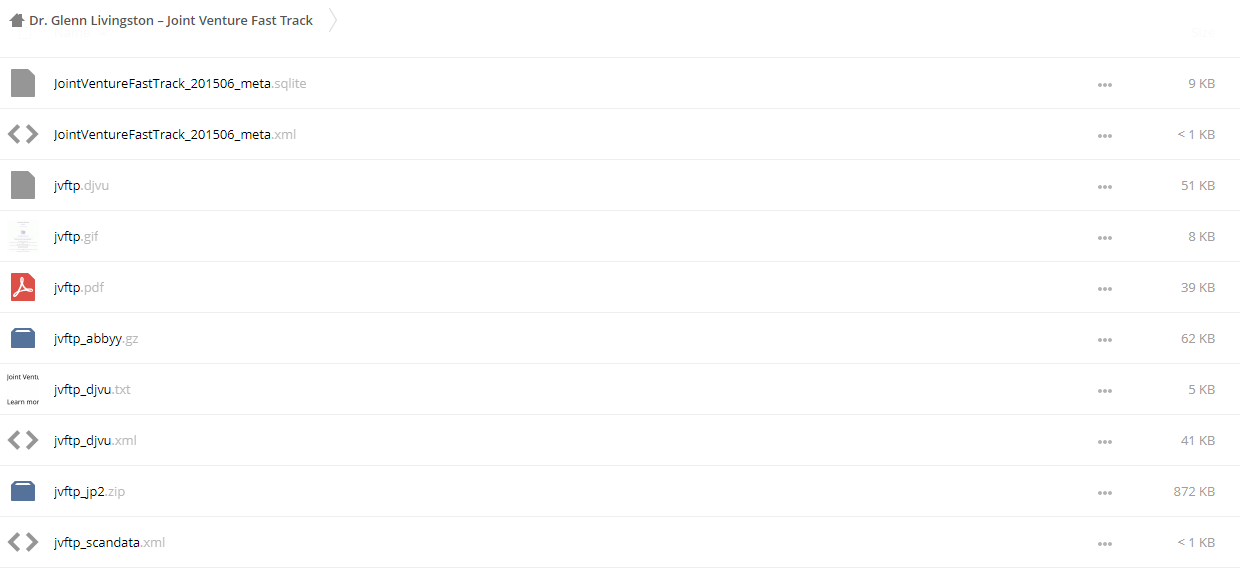Dr. Glenn Livingston appears to be meticulously reviewing a series of documents and PDFs on his computer screen. The screen displays a list of digital files, each with varying sizes and formats, related to a project possibly named "Joint Venture Fast Track." The topmost document bears Dr. Livingston's name, indicating that he is looking through different PDFs and other documents.

The first file listed is a grey document titled "Joint Venture Fast Track Meta," showing its size all the way to the right. Below this, another file, also named "Joint Venture Fast Track," is listed as less than a kilobyte with a left-right arrow icon next to it. Following this, a larger file named "JV FTP DJView" is 51 kilobytes in size. There is also an 8-kilobyte GIF image.

Further down, a PDF file is marked at 39 kilobytes titled "JV FP Abby." Another entry, "JV DFP DJView," is listed as text with a file size of 5 kilobytes. The same file appears again in an XML format with a size of 41 kilobytes.

The document names and file sizes are predominantly grey, set against a white background, with few elements in shades of blue and red, giving the interface a minimalist look. These documents possibly contain patient information or details about joint ventures in the medical field that Dr. Livingston is currently working on.